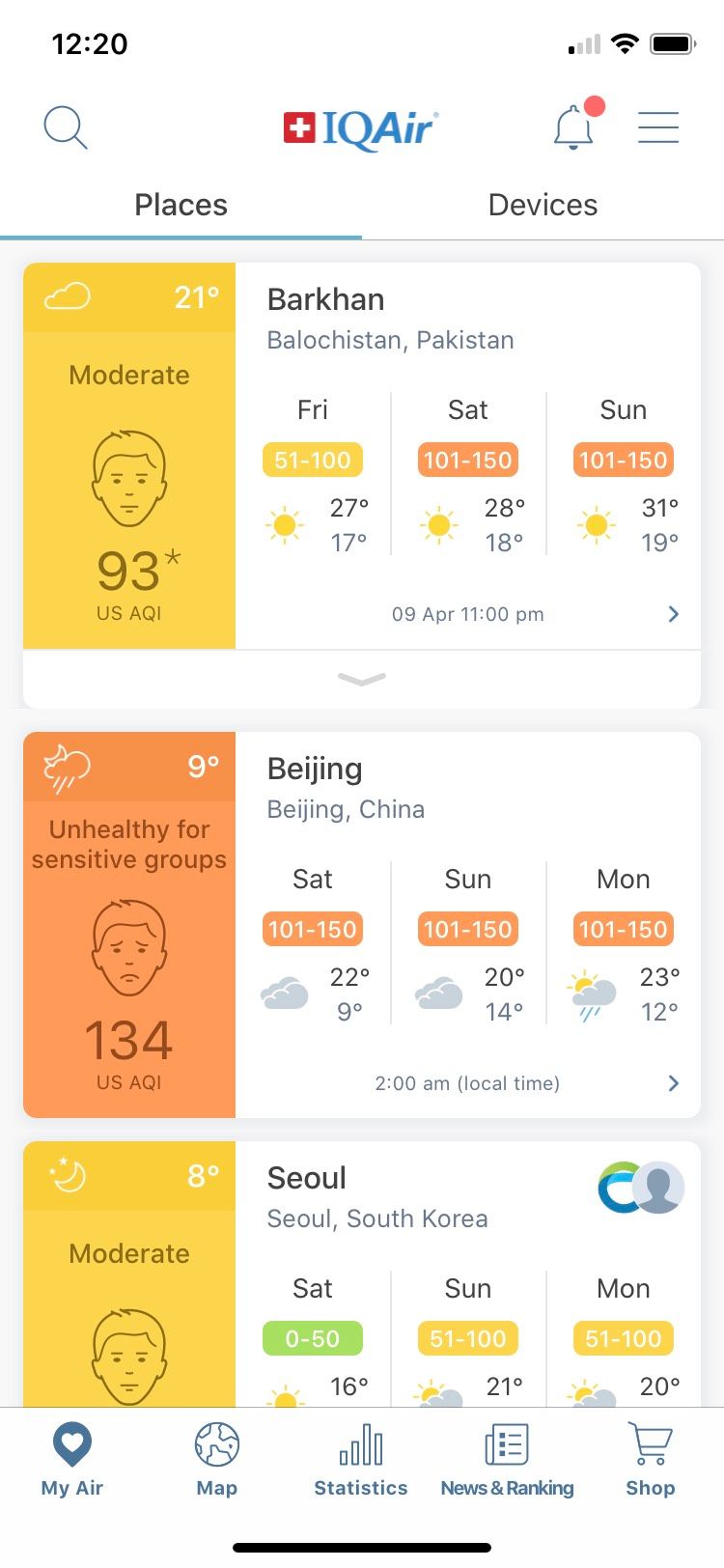In this image captured from a cell phone screen, the "IQ Air" app is displayed. At the top of the screen, tabs for "Places" and "Devices" are visible, with a blue line under "Places," indicating that this tab is currently selected. The screen’s header showcases weather information for multiple locations: Barkhan, Beijing, and Seoul, with the option to scroll for more.

For Barkhan, Pakistan, the app shows a moderately polluted air quality with an AQI (Air Quality Index) of 93 inside a yellow box. The weather conditions are represented by a cloud icon, with the temperature being 21 degrees Celsius. Additionally, there is a child-like face displaying a neutral expression indicating moderate air conditions.

In Beijing, the air quality is marked as unhealthy for sensitive groups, indicated by an orange box and a frowning face, showing the AQI at 134. The temperature in Beijing is 9 degrees Celsius.

For Seoul, the app indicates an AQI categorized as moderate, with a reading of 8 degrees Celsius. The air quality is represented by a neutral face, showing that the air quality is acceptable but could be better.

The overall visuals include icons for weather conditions (such as clouds), temperature readings, and expressive faces to quickly convey the quality of the air.